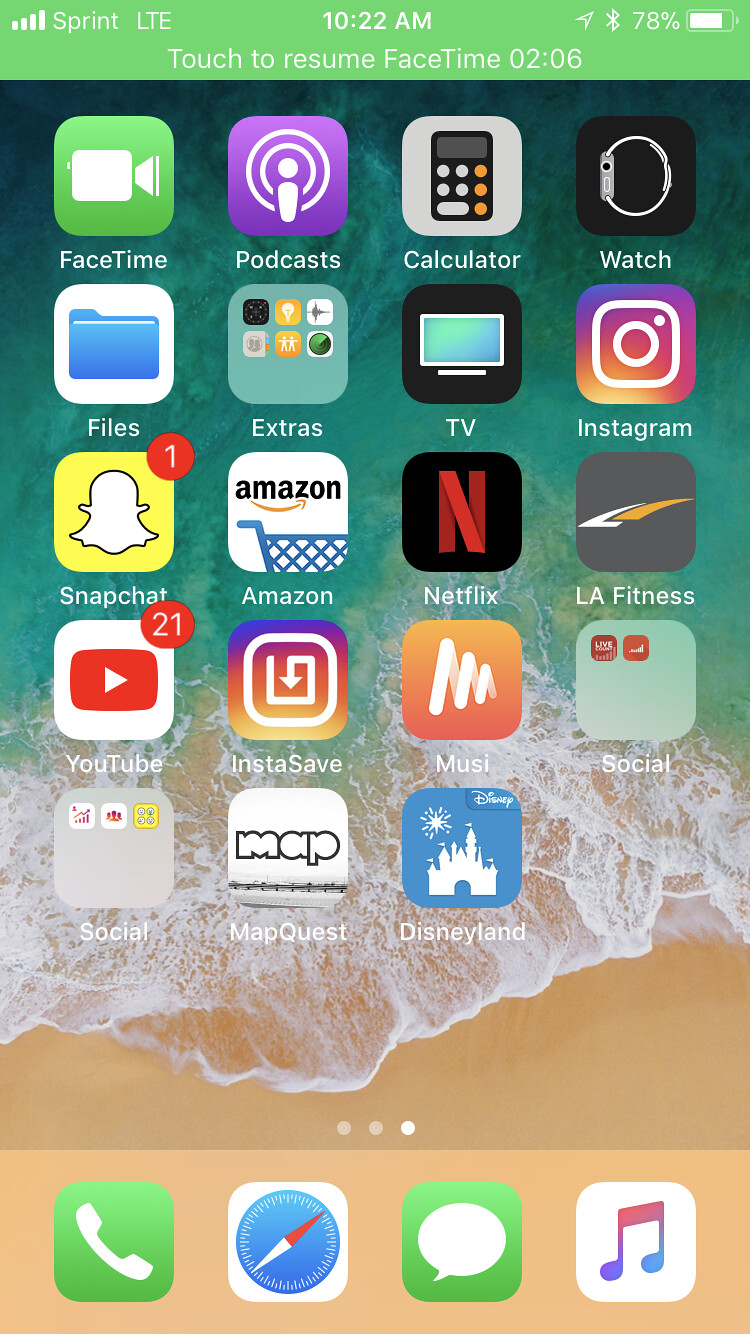This image is a detailed screenshot capturing a beachfront scene with an overlay of a mobile device's home screen. The primary visual feature is a picturesque beach with tan-colored sand giving way to a gradient ocean. The ocean transitions from a white frothy surf to an aqua hue and culminates in a darker aqua at the horizon, accentuating the waves' tips in white. This entire scene is encased within a rectangular frame.

At the top of the screenshot, there's a green status bar indicating the device's status: it shows "Sprint LTE," the current time "10:22 AM," the battery level "78%" accompanied by a battery icon, and a notification reading "Touch to resume FaceTime, 02:06" beneath the time. A FaceTime icon is positioned in the upper left corner. 

Below the status bar, the home screen is arranged into four rows of four icons each:

- **Row 1:** FaceTime, Podcasts, Calculator, Watch.
- **Row 2:** Files, Extras, TV, Instagram.
- **Row 3:** Snapchat, Amazon, Netflix, LA Fitness.
- **Row 4:** YouTube, Instasave, Muse, Social.

Additionally, there are three more icons: Social, MapQuest, and Disneyland.

At the bottom of the home screen, there are four essential icons for quick access: Phone, Maps, Chats, and Music.

Noteworthy are the three small red circles located on the sand between the status bar and the main set of icons, blending from the tan color of the sand to white, providing a subtle color transition.

This meticulous description captures both the serene beauty of the beach scene and the structured chaos of the mobile device’s home screen grid.